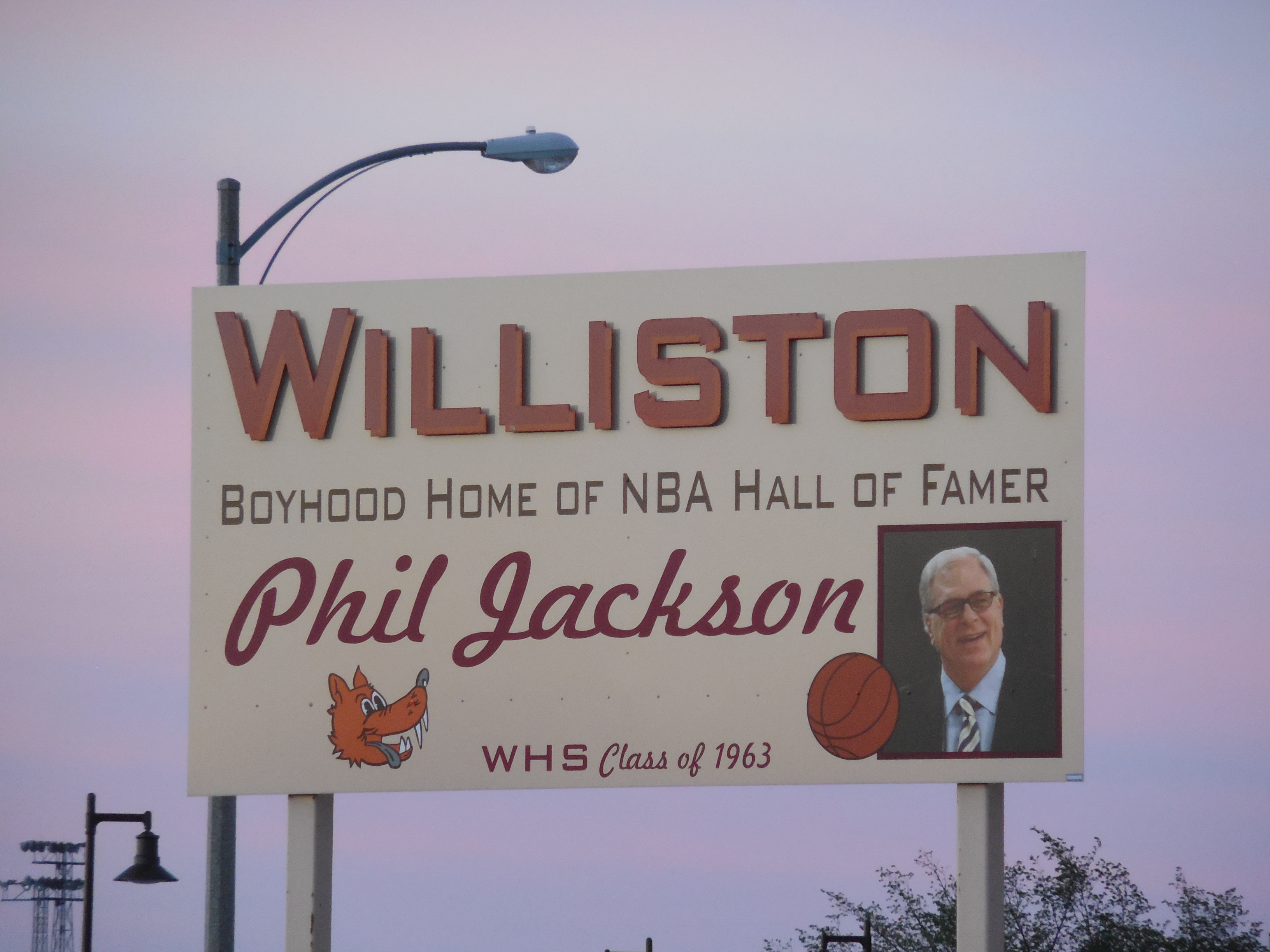The image features an outdoor setting at dusk with a central white billboard as the main focus. The billboard prominently displays the text: "Wilson, Boyhood Home of NBA Hall of Famer Phil Jackson. Wilson High School Class of 1963." The top text is in a light salmon brownish-red, with "Phil Jackson" written in red cursive underneath. Positioned to the bottom right of the sign, there's a picture of an older gentleman, likely Phil Jackson, accompanied by a basketball. On the bottom left corner of the sign, there is a cartoon logo of a wolf, marking the school logo. Surrounding the billboard are various street features: lamps and streetlights to the left, power lines, and some trees on the bottom right. The sky in the background is transitioning into night, casting a darker, early evening ambiance over the scene.